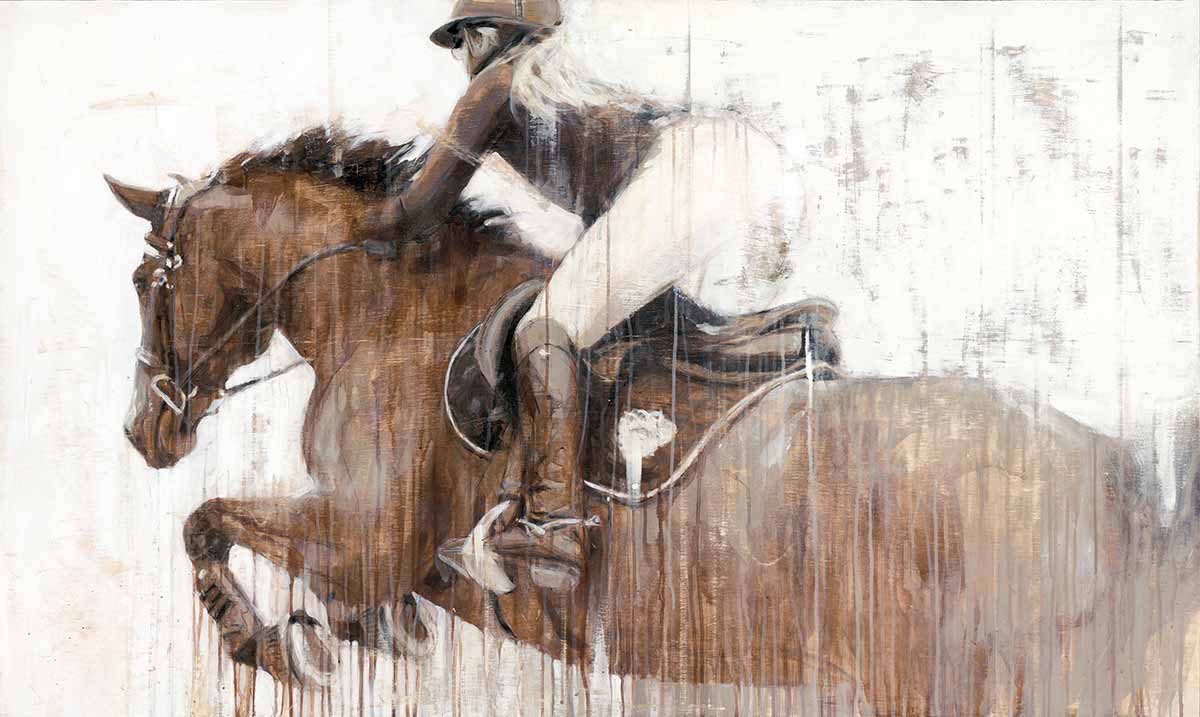This is a detailed color illustration of a horse derby rider, specifically a female jockey, on a brown horse in mid-jump, set against a white background. The horse's front legs are tucked underneath it, hooves off the ground, and a brown saddle with a brown saddlecloth is visible. The jockey, looking to the left, is standing high in the stirrups, squatting above the saddle, giving the impression of guiding the horse over an obstacle. She is dressed in white riding pants and knee-high brown boots with small spurs. Her attire includes a long-sleeved brown silk shirt and a brown helmet with a chin strap. Additional details such as her long hair flowing and the horse's brown mane in the reins add to the dynamic motion of the scene. The image is overlaid with distress lines and marks, giving it a vintage and worn appearance.